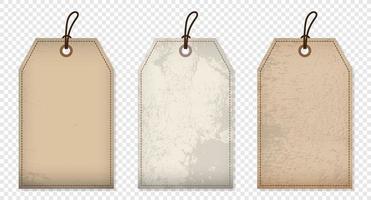The image depicts three suitcase tags placed in a row against a subtle blue and white checkered background. Each tag has a nearly rectangular shape with the top corners cut diagonally. They feature small holes at the top, through which little strings are attached, enabling them to be tied to luggage. The leftmost tag is beige and appears to be made of leather, with a stitched border that suggests cloth texture. The middle tag is gray, also with a stitched border and the same string attachment. The rightmost tag is beige like the first one but shows some scratches on its surface, adding a worn texture.